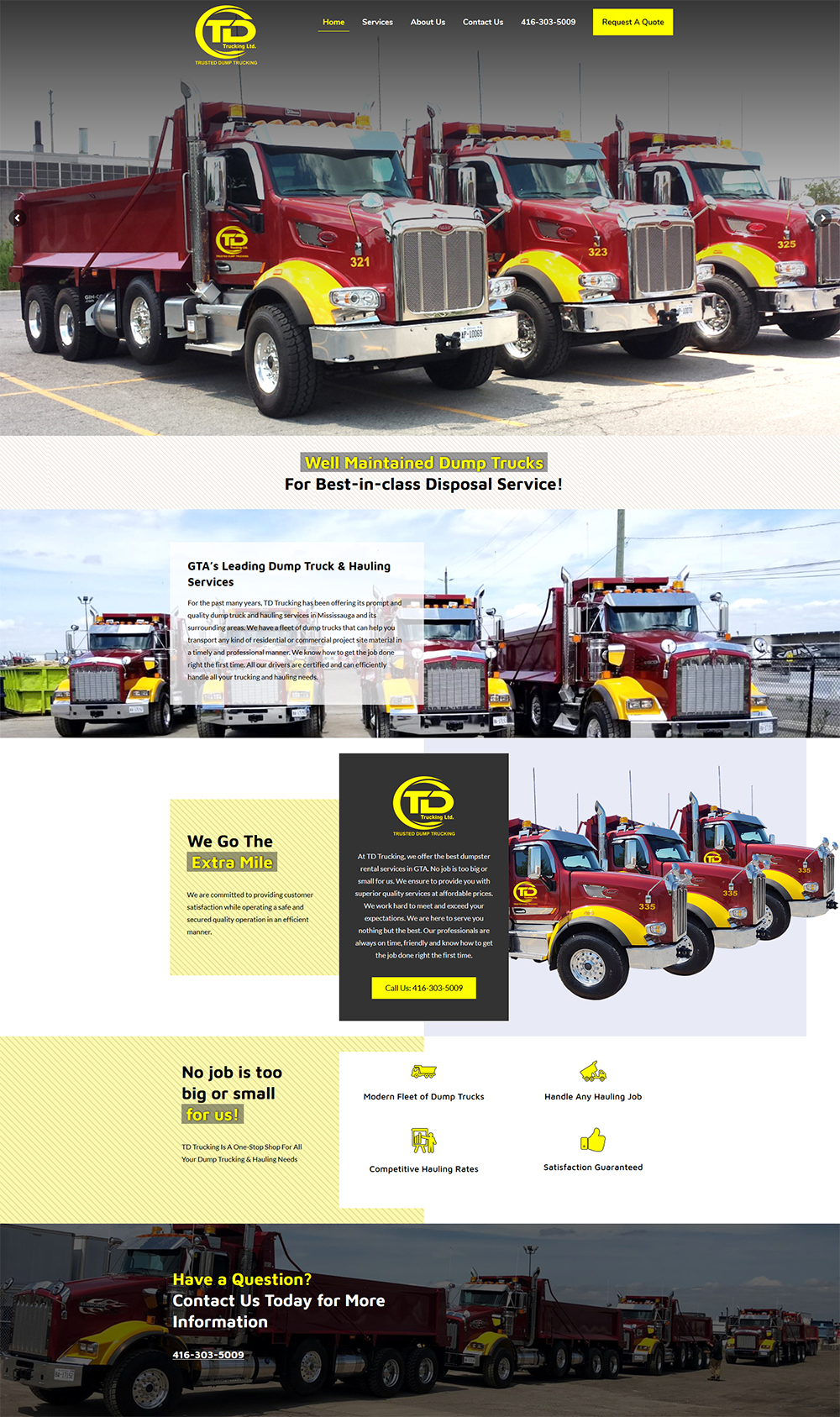**Caption:**

A montage of images showcases a fleet of well-maintained, red dump trucks, featuring three trucks with prominent big tires and yellow accents on the upper part above the front tires. These dump trucks, emblazoned with the initials "TD" in bold yellow letters, represent best-in-class disposal services. Another frontal shot reveals four dump trucks lined up, accompanied by a header proclaiming "GTA's Leading Dump Trucks and Hauling Services." This section also includes a detailed drawing where the trucks are displayed side-by-side at an angle, with the "TD" logo prominently displayed.

Adjacent to these visuals is a yellow box with a motivational tagline, "We go the extra mile," followed by another yellow banner confirming that "No job is too big or small for us." Below these messages, four icons are presented—a truck, a numeral "2," another icon, and a thumbs-up—each accompanied by relevant text details. The lower section features an additional ad banner urging viewers to contact the company for more information, along with a visible phone number. The phrase "Have a question?" stands out in yellow, and the background reveals more trucks subtly darkened but still discernible, reinforcing the company's extensive fleet and capabilities.